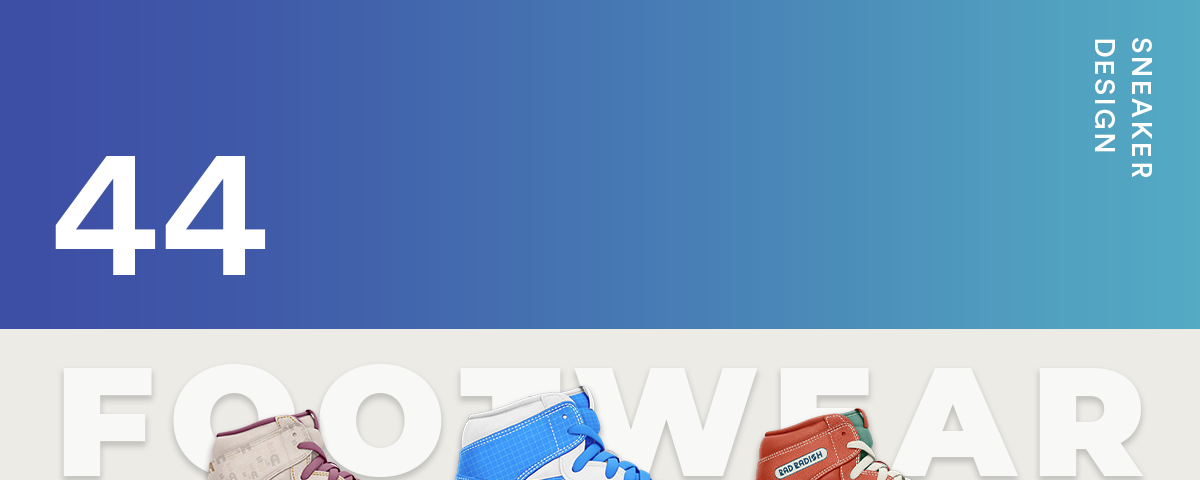The image appears to be a truncated page, likely from a catalog or online catalog, depicting a vibrant horizontal strip transitioning from deep blue on the left to turquoise on the right. On the left side of the strip, the number "44" in bold white letters stands prominently. On the upper right-hand corner, "Sneaker Design" is inscribed vertically from right to left, over a more turquoise background. Below this, a distinct gray bar displays the word "Footwear" in three-dimensional white lettering. Positioned in front of this bar are the partial tops of three high-top sneakers. The first sneaker, on the left, is beige with brown laces. The middle sneaker is white with blue trim and blue laces, while the one on the right is orange-red with white laces and a green tongue. This image segment seems to advertise different sneaker designs, yet the remaining portion needed for complete context is not visible.